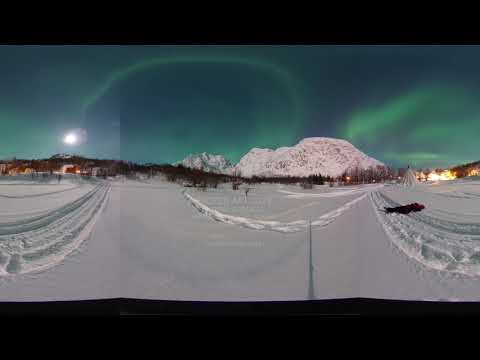This panoramic image captures a mesmerizing winter night scene, dominated by a vast, snowy landscape under a sky illuminated by the Northern Lights. The foreground is blanketed in untouched snow, crisscrossed by distinct tracks, possibly from a snowmobile. On the right side of the image, a person is seen lying in the snow, perhaps gazing up at the vibrant aurora that paints the sky in shades of green, blue, and turquoise. The middle ground features a small village with clusters of houses or buildings, emanating warm lights that cut through the cold, dark night. A triangular structure hinting at a teepee is faintly visible among the buildings, adding a mysterious element to the scene. To the far left, there are more distant buildings and a hazy sun or moonlight above the horizon, casting a subtle glow. In the background, a tall hill and distant snow-capped mountains frame the image, lined sparsely with trees. The image is bordered by black bars at the top and bottom, providing a cinematic feel to this serene and magical winter night.